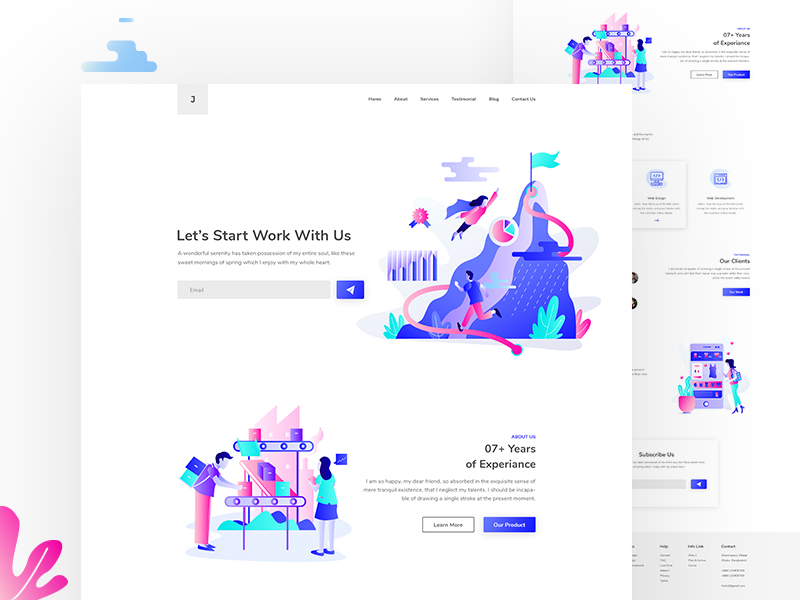On the page, there's an image of a dynamic, whimsical website interface. At the top, a vibrant banner displays the slogan "Start Working With Us," encouraging visitors to engage. The header features an input bar for entering information accompanied by a prominent blue button. 

Dominating the image is an artistic depiction of a woman soaring upwards with a cape, symbolizing empowerment, while a man runs alongside. This scene is set against a backdrop of blue and purple mountains, creating a sense of aspiration and ambition.

Further down, there's text mentioning "7+ Years of Experience," though it's barely legible due to blurriness. Adjacent to this, a white button with black font invites users to "Learn More," while a blue button labeled "Our Product" stands out.

Below this, the image portrays a man and a woman at an assembly line, diligently working amidst boxes, symbolizing productivity and teamwork.

The bottom section of the image reiterates "7+ Years of Experience" and "Our Clients." The overall design is colorful, utilizing shades of blue, pink, green, white, black, and gray, creating an engaging and professional atmosphere.